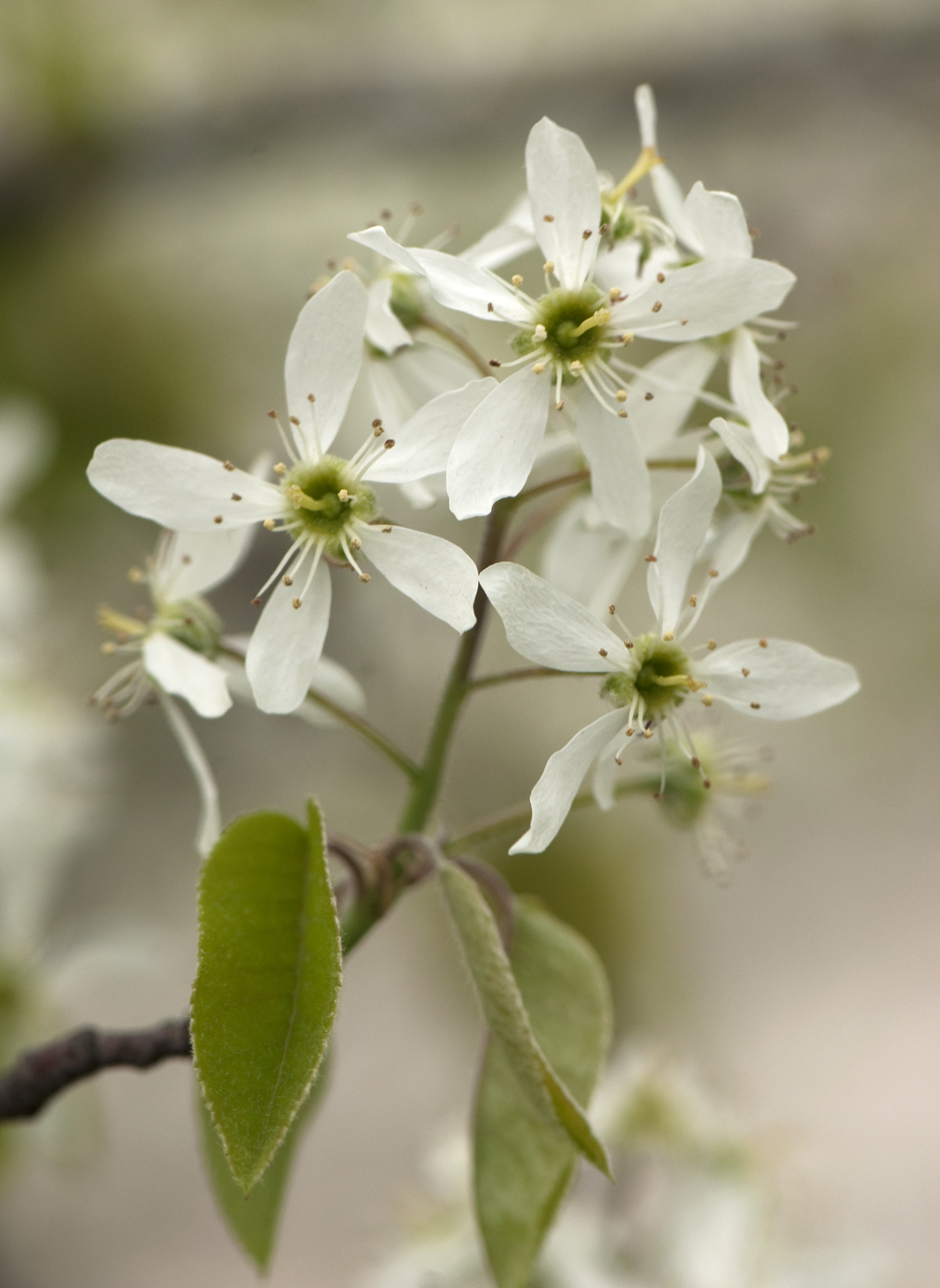This close-up photograph features a cluster of small, likely prunus family, white flowers adorning the tip of a knobbly brown tree branch that curves towards the left side of the image. Each flower has five delicate white petals surrounding a light green center, from which long, slender stamens extend with brown-tipped anthers. The cluster appears to contain between six to ten flowers. Nestled just beneath the blossoms are a few oval-shaped leaves with pointed tips and serrated edges, adding a vibrant green contrast to the composition. The background is a soft blur of white, green, gray, and brown hues, drawing focus to the intricately detailed flowers and leaves in the foreground. This image captures the delicate balance and beauty of nature in bloom.